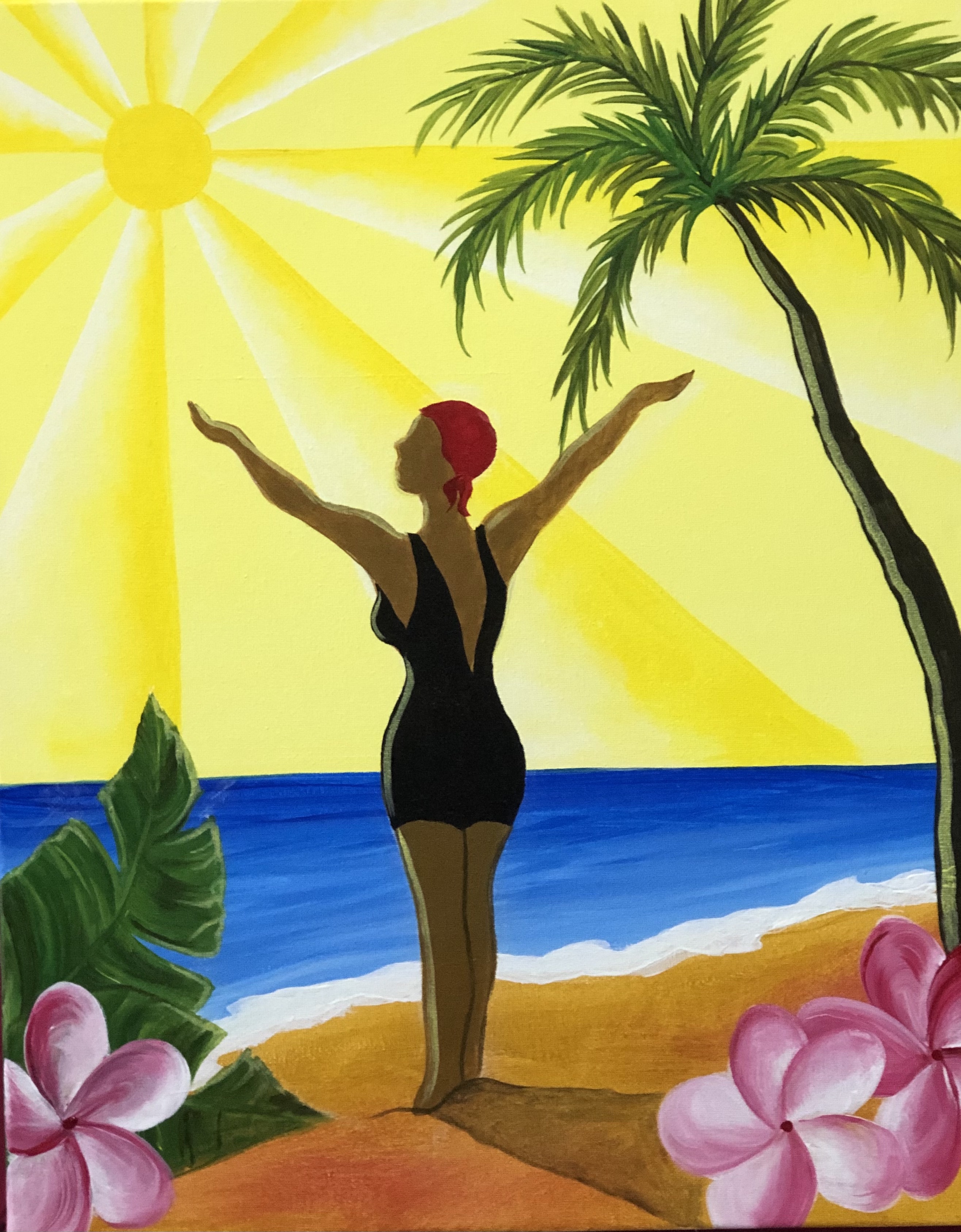This painting captures a serene beach scene with a woman standing on the sandy shore, framed by nature's beauty. The woman, dressed in a black one-piece swimsuit with a deep V, has her arms outstretched towards the vibrant sky, embracing the warmth of the sun. A red bathing cap adorns her head. The backdrop features a stunningly blue ocean with white waves gently crashing onto the shore. The sky is dominated by a radiant sun, whose yellow and white rays cascade down, illuminating the entire scene with a sunshiny glow. To the right of the woman, a tall palm tree angles gracefully towards the water. The foreground is enriched with lush greenery, including a large leafy fern on the left and several vibrant pink flowers that evoke a tropical, Hawaiian vibe. The overall composition is colorful and filled with light, capturing a moment of peaceful reflection and joy.